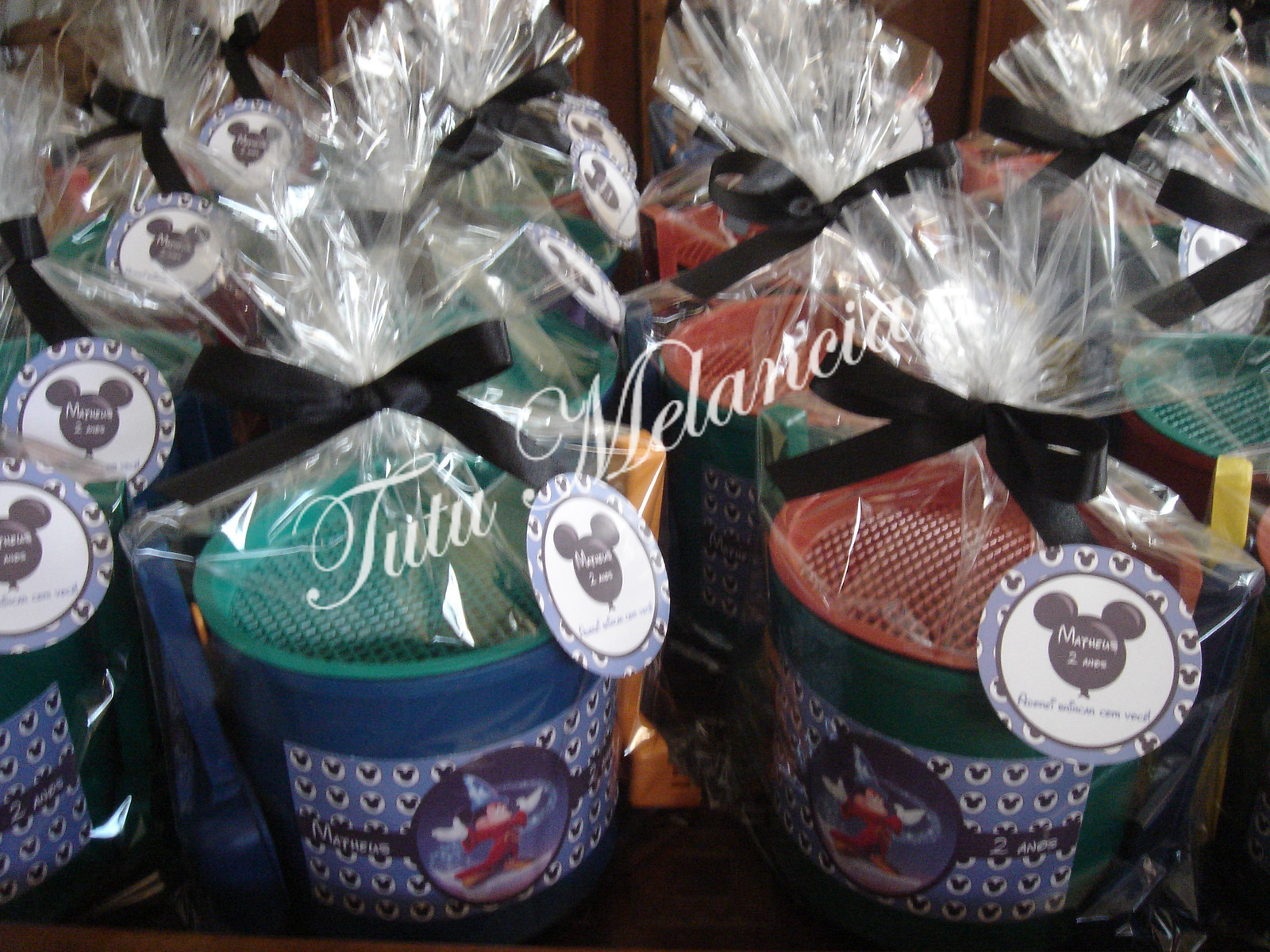This is a detailed photograph in horizontal orientation, showcasing a large number of decorative buckets arranged in several rows that stretch deep into the image, possibly four or five buckets deep. The primary colors of the buckets are blue and green, with some buckets featuring red lids and others green. Each bucket is meticulously wrapped in clear cellophane and adorned with a black bow tied at the top. 

In the foreground, a light blue circle prominently displays an image of Mickey Mouse dressed in his iconic magician outfit from Fantasia, complete with a blue hat decorated with white stars, a red robe, and white gloves. Around Mickey, there are subtle images of Mickey Mouse head logos. Each bucket also features a tag with a white background and a black Mickey Mouse head logo, which includes round ears and a round head, along with names written in a white, handwritten-style text. The tag on one of the front buckets reads "Matthias" with the number two beneath it. Additionally, a watermark reading "TUTU MELANCIA" is visible in the middle area of the photograph.